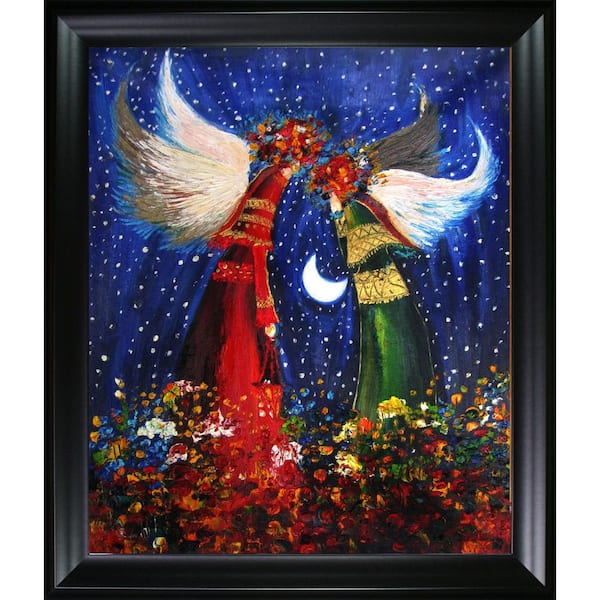The image is a framed painting set in a thick, black, beveled frame that appears to be either oil or acrylic. This whimsical and colorful scene depicts two angels with white feathery wings standing in a vibrant flower garden under a night sky. The garden is abloom with myriad red, yellow, blue, orange, and green flowers. 

The angel on the left wears a flowing red robe adorned with gold fringe around the shoulders and cuffs and has their hands at their sides. The angel on the right wears a similar dress in green, also with gold fringe, and has their hands raised by their face. Both angels have their heads adorned with an abundance of flowers in red, orange, and blue, so much so that their faces are obscured.

They are facing each other towards the center of the painting, with a crescent moon and twinkling stars shining in various shades of dark blue in the sky between them. The backdrop around their wings is slightly lighter blue, adding a mystical, ethereal glow to the scene.